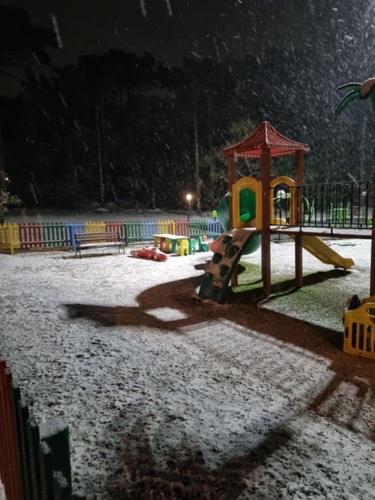This image is a detailed nighttime color photograph of a children's playground, brightly illuminated from a light pole outside of the camera's view, casting light primarily on the upper right side. The ground appears to be covered in a thin layer of snow or possibly sand, creating an ambiguous texture. A defining feature of the playground is a multicolored fence painted in a repeating pattern of green, blue, yellow, and red that encloses the area. Central to the scene is a yellow slide with red pillared railings, a red roof, and an adjacent small green climbing structure, all part of a larger playground apparatus with a walkway above. Additional park features include a couple of tables, a bench in the background, and the overall area of the park is approximately 100 meters by 100 meters. The setting and design elements evoke a subtle oriental style, suggesting it might be located somewhere in Southeast Asia.